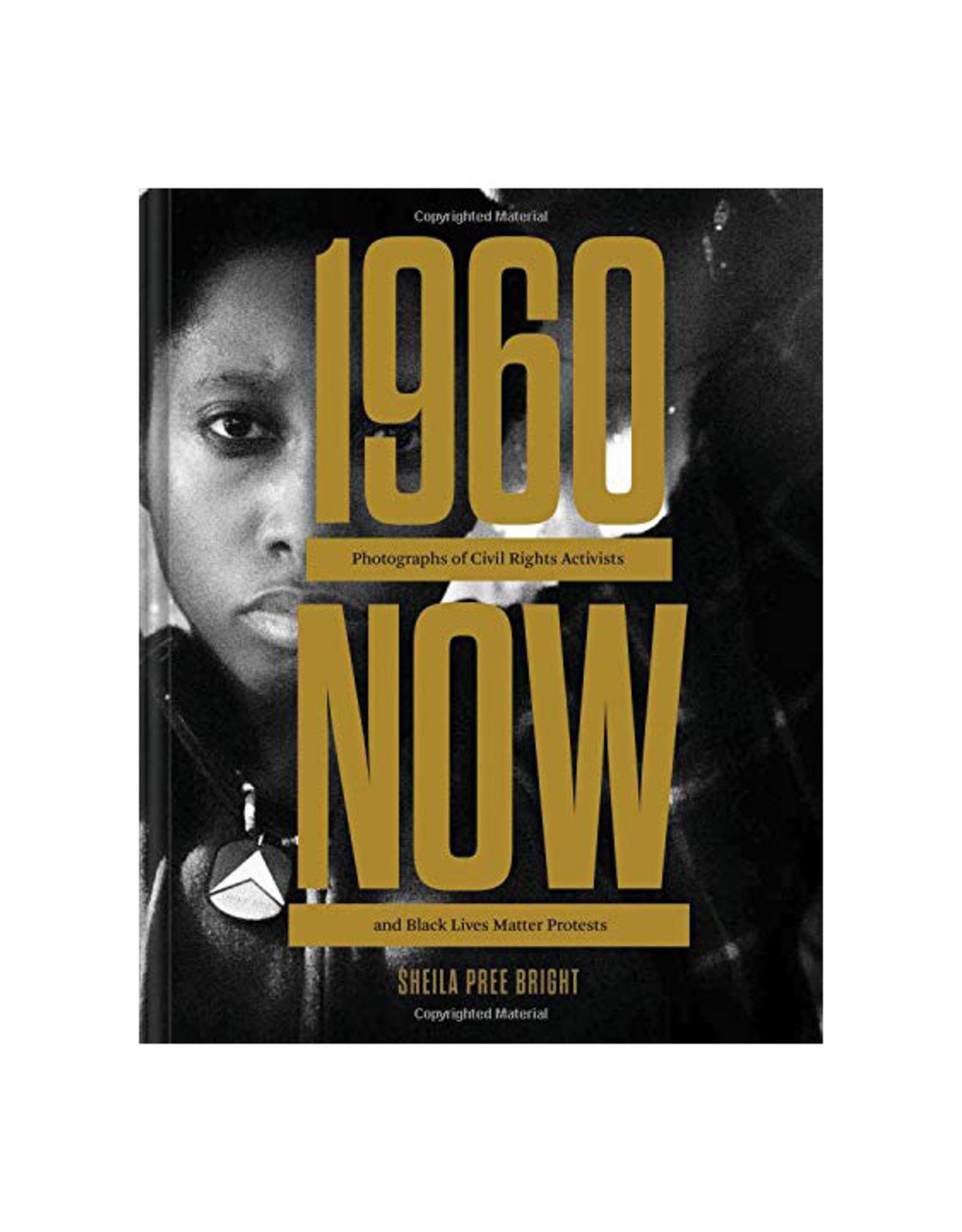The cover is predominantly black and white with gold and brown text. At the top, it reads "copyrighted material." Below that, in bold and large gold letters, is "1960," underlined by a thick brown bar. Inside the bar, in black-to-dark gray text, it says "photographs of civil rights activists." Beneath this, the word "NOW" stands out in bold brown font. Following "NOW," another brown block contains the text "In Black Lives Matter protest" in black font. At the bottom, written in a brownish-gray color, it states "Sheila Pree Bright," along with "copyrighted material." Covering the background is an image of a Black woman, who is raising her arm as she looks directly at the camera. She wears a pendant shaped like an oval with an upside-down V inside it, distinct in its white color against the darker palette. The overall format suggests it is a book cover, upright in a vertical rectangle style, combining an illustration and a realistic photograph.